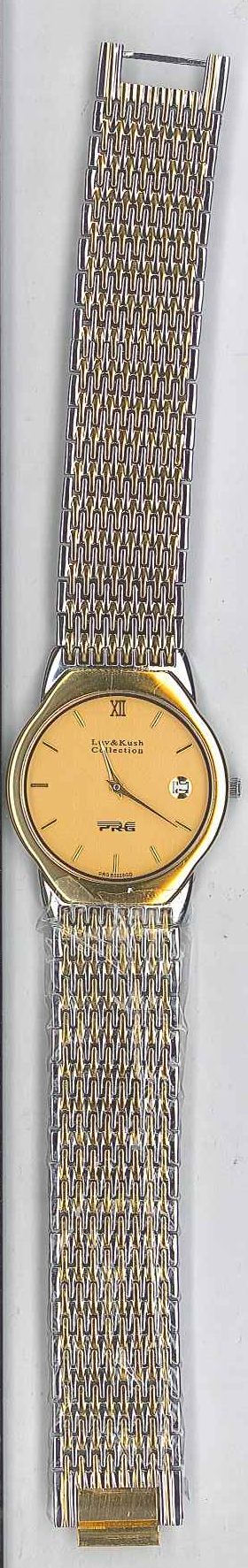This detailed product image features a vertically-oriented, brand-new wristwatch. The photograph, rectangular in shape, showcases the watch centrally against a light grey background without any additional text or overlay. The watch itself has a slightly curved alignment, with the top curved to the right and the bottom to the left. The band is an interlocking chain design combining gold and silver tones. The top of the band has a silver clasp, while the bottom features a gold-toned clasp for securing the watch. The circular watch face is predominantly light gold, encircled by a darker silvery-gold bezel. It displays Roman numerals with the hour markings in dashes, except for the numeral XII at the top. The time shown is twenty minutes past eleven. There is a small white rectangle at the three o’clock position, potentially an in-face date display. The peach-toned interior of the face and the overlying Roman numerals enhance the elegant appearance, making the timepiece appear luxurious and pristine.